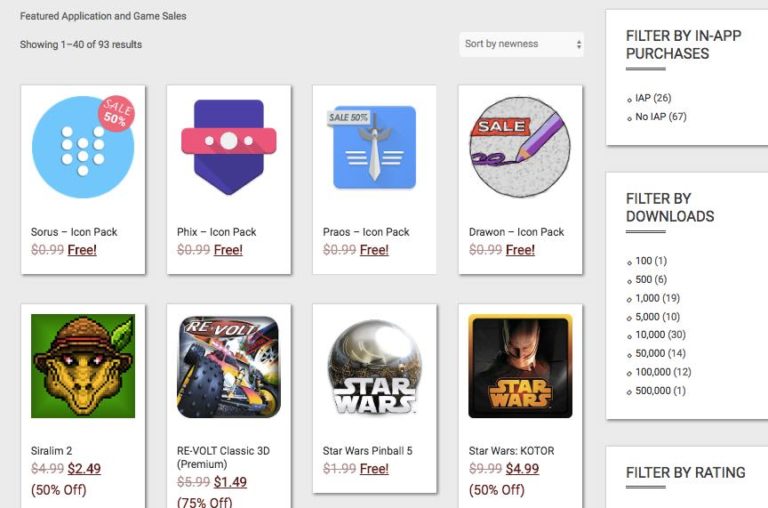Screenshot of App Store Page Featuring Application and Game Sales

The image is a screenshot from an app store page, characterized by a light grey background and multiple white boxed sections containing information and images. 

At the top left of the screenshot, the text "Featured Application and Game Sales" is prominently displayed, followed by "Showing 1 to 40 of 93 results." Moving horizontally to the right, there is a dropdown menu labeled "Sort by Newness" with up and down arrows, indicating various sorting options.

On the right-hand side of the image is a vertical column consisting of three white boxes:
1. The topmost box bears the bold, capitalized heading "FILTER BY IN-APP PURCHASES" with a small underline. It lists two bullet points: "IAP (26)" and "No IAP (67)."
2. Below that, the second box is titled "FILTER BY DOWNLOADS." It offers eight options sequentially ranging from 100 to 500,000 downloads.
3. At the very bottom right corner, there's a partial view of another box titled "FILTER BY RATING."

Returning to the main screen, the central section showcases two horizontal rows of application icons:
- **First Row**:
  1. **Soros Icon Pack**: Depicted by a blue circle with a red "Sale 50% Off" badge, currently free.
  2. **Fix Icon Pack**: Featuring a purple shield with a pink diagonal line and three white dots, also free.
  3. **Preyos Icon Pack**: Illustrated by a blue square with a sword and three white horizontal lines, free as well.
  4. **Draw On Icon Pack**: A circle with "Sale" text and a purple pencil, also marked free.

- **Second Row**:
  1. **Cyrillim 2**: Represented by a green square with a crocodile wearing a hat icon.
  2. **Revolt Classic 3D**: Displaying what appears to be a car icon.
  3. **Star Wars**: Two icons, one detailed, and the other a simple yellow text on a square background.

Each icon pack and app comes with distinct visual markers, providing a detailed overview of their appearances and current sales status.